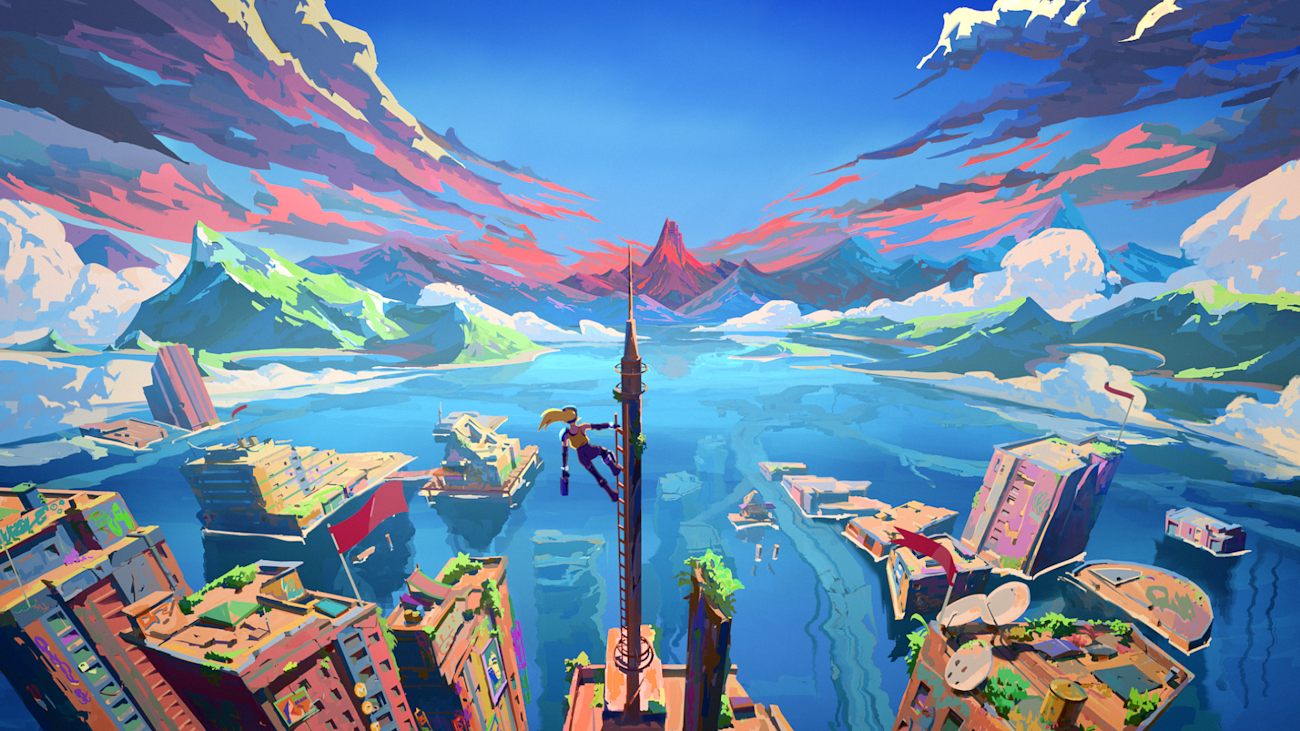This vibrantly painted, cartoon-like image portrays a fantastical, flooded cityscape viewed from a high vantage point, with a subtly curved perspective in the foreground. At the very center stands a tall, thin skyscraper-like tower. Clinging to the left side of this tower is a woman adorned in blue and yellow clothing, with a long blonde ponytail, seemingly trying to escape the submerged city below. The flooded city consists of multi-story buildings that exhibit brown tones with blue windows, some painted in pink and blue hues. Vegetation and satellite towers are visible atop these buildings, resembling park-like settings. A burgundy flag flutters amidst four of the underwater buildings on the left side of the image, while three more are partially submerged on the right. In the distant background, lush green mountains draped in white clouds span the sides of the image, contrasting with a striking blackish-red mountain at the center, which is encircled by ominous gray clouds at its peak. Pink mountains and icebergs further accentuate the fantastical nature of this otherworldly scene.